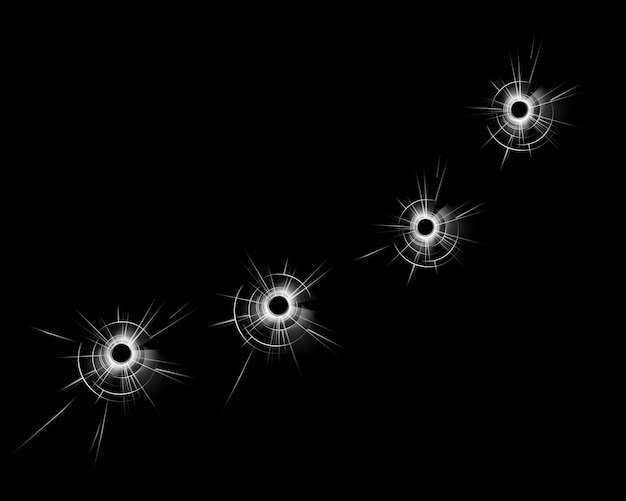The image depicts a solid black background featuring four white circular illustrations resembling bullet holes in glass. These bullet-hole-like shapes, composed of white circles and radiating lines, are arranged in a roughly diagonal line stretching from the bottom left corner to the upper right corner. The first hole is located in the bottom left, the second slightly to the right and up, the third further to the right and slightly higher, and the last one in the upper right corner. The white illustrations are bright and stand out sharply against the black background, giving the impression of shining light. The overall composition is in landscape orientation, wider than it is tall, with no bullet holes appearing in the top left or bottom right corners.